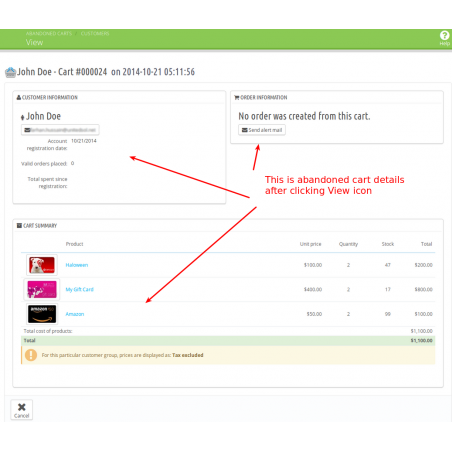This is a screenshot of a website interface, specifically displaying details of an abandoned shopping cart. A green banner atop the page features the word "View" in white text on the left, with a white circle containing a question mark labeled "Help" on the right. There is some unreadable text above the "View" button due to blurriness.

In the main section below the banner, it reads: "John Doe cart 000024 on 2014-10-21 5:11:56." Further down, the customer information section details "John Doe" and lists an account registration date of "10-21-2014". It notes that zero valid orders have been placed and shows the total spent since registration as zero.

Under "Order Information," it indicates that "No order was created from this cart" and includes an option to "Send alert mail."

At the bottom of the page, in the "Cart Summary" section, items are listed with the corresponding details: 
- "Halloween" with a unit price of $190 and an unclear quantity of $22.
- "My Gift Card" with a unit price of $480, stock of $47, and a subtotal displayed as $200.
- "Amazon" with a unit price of $93, quantity of 2, and an unclear total of $800.
- Additional unclear totals of $100, combining to a final total of $1100.

A note at the bottom specifies: "For this particular customer group, prices are displayed as tax excluded."

Red arrows have been annotated pointing to the sections labeled "Customer Information," "Send alert email," and "Cart Summary." Additionally, red text has been added to the image stating: "This is the abandoned cart details after clicking the View icon."